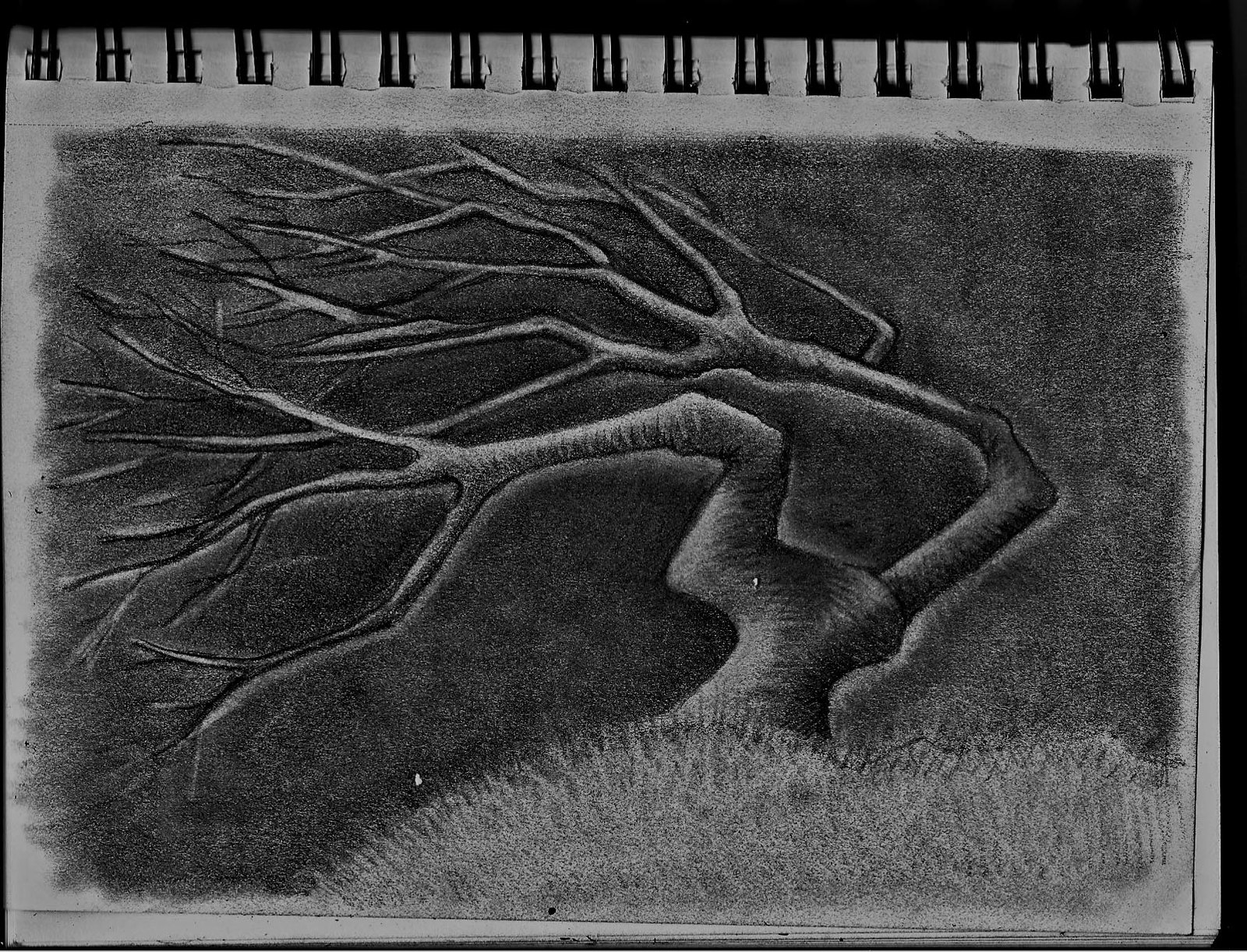This is a detailed photograph of an artist's spiral-bound sketchbook, opened to a page showcasing a meticulously drawn tree. The black and white pencil sketch captures a tree with its branches dramatically bent backwards, as if struggling against a powerful wind. The detailed application of pencil shading renders this artwork in a strikingly realistic manner, with the tree's numerous branches and leaves depicted as if they are being blown intensely towards the left side of the page. The tree stands on a grassy hill, its trunk and foliage intricately shaded to create a three-dimensional effect. The dark background enhances the scene, suggesting a stormy, windy night. This evocative drawing, free from any textual annotations, makes full use of the sketchbook’s space and cleverly utilizes the spiral binding to extend the depth and dimension of the composition.